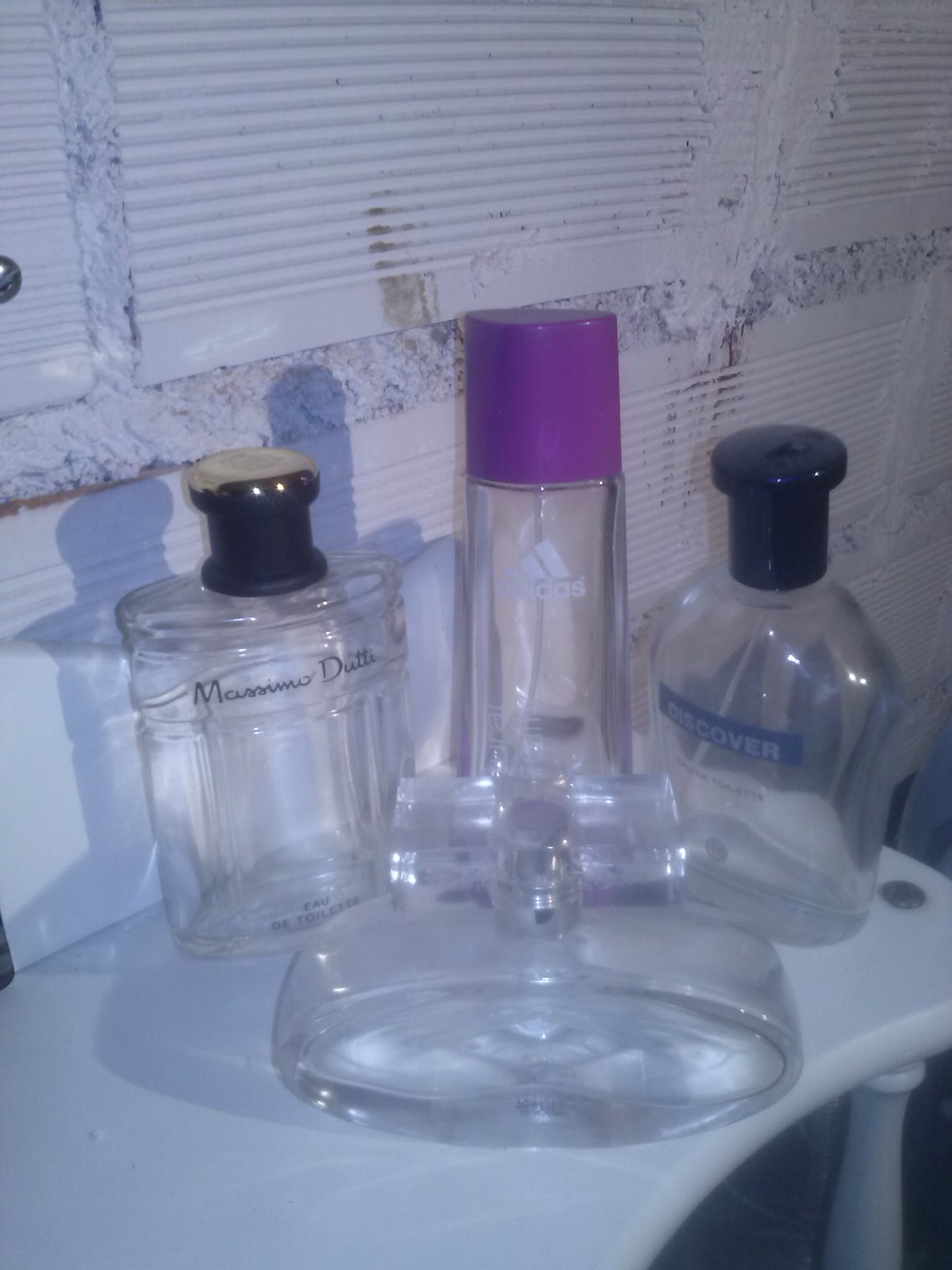The image is a detailed, close-up color photograph in portrait mode, showcasing five seemingly empty glass perfume or cologne bottles arranged on a flat white surface, likely a table or vanity, with a white wall serving as the background. From left to right, the bottles are positioned as follows: an elegant Massimo Dutte bottle with a black and gold cap, followed by a tall Adidas bottle with a distinctive purple spray cap. To the right of the Adidas bottle is a Discover bottle with a black cap. In the foreground is a smaller, squat, oval-shaped bottle with a cross-shaped glass stopper, and behind it, a small square bottle. The bottles, arranged in a visually appealing manner, are set against a backdrop of textured wallpaper featuring white, blue, and pink hues.